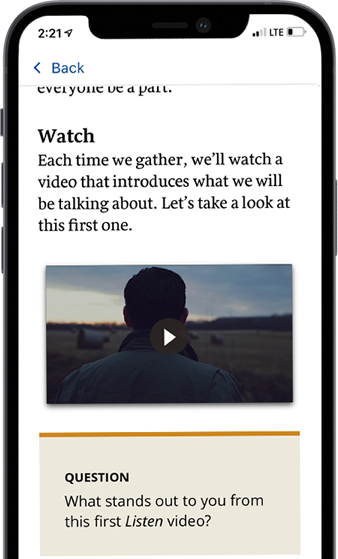In the image, a cell phone, which appears to be an iPhone, displays a screenshot of an app interface. The top left corner features a blue "Back" button with a capital "B". The status bar reveals a weak LTE signal and a nearly depleted battery, with roughly 25% remaining. The phone itself has a black trim, a silent button on the left side, and volume control buttons above it.

The main content of the screen starts with the text "Everyone be a part." Below that, there's a section labeled "Watch" with the description: "Each time we gather, we'll watch a video that introduces what we will be talking about. Let's take a look at the first one."

A play button overlays an image of a man, seen from behind, who is wearing a coat and standing in an open area with visible greenery. Beneath the video section, there is a query labeled "Question:" followed by, "What stands out to you from this first listen?" with "listen" italicized. This indicates the prompt for the viewer to reflect upon after watching the video. The overall background of the app interface is white.